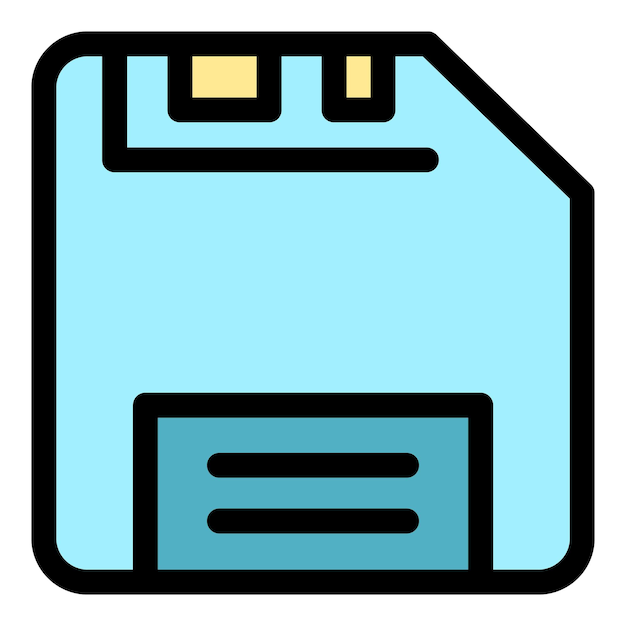The image showcases a highly stylized and zoomed-in cartoon depiction of a floppy disk against a white background. This playful illustration features a square shape with rounded corners, distinguished by a deliberate notch taken out of the upper right corner. The disk predominantly showcases a light blue color palette with a darker blue section at the bottom, accented by black stripes. In the upper part of the disk, small yellow rectangles add a touch of detail. The entire image is outlined with thick black lines, providing a bold and easily recognizable appearance. The overall design is simple and clipart-style, with no text present, making it a quick and effective visual reference. Interestingly, the disk drive area at the bottom portrays a friendly face, with yellow rectangles as eyes and a small black smile, imparting a whimsical, nostalgic charm suitable for both children and adults. This description paints a detailed picture of a cheerful and recognizable floppy disk icon, blending functionality with a touch of character.